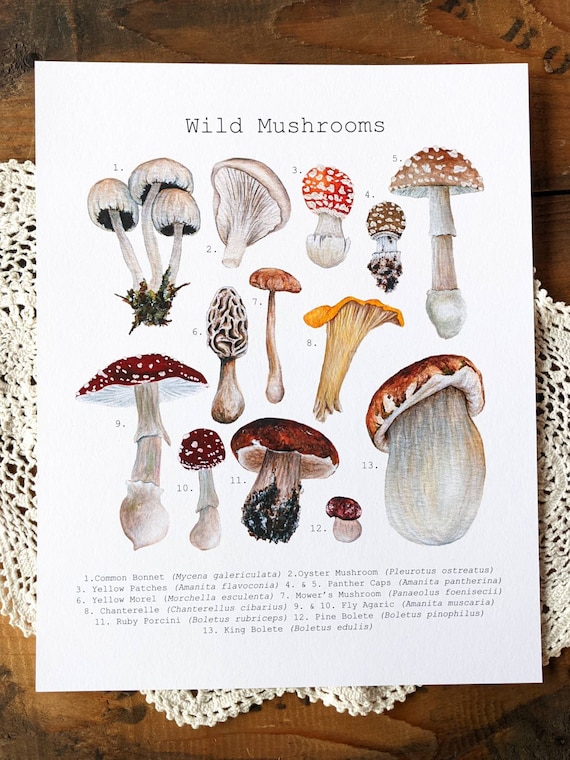The image captures a detailed poster titled 'Wild Mushrooms,' set against a white doily lace material on a rustic wooden table. The poster features a clean, white backdrop with the title 'Wild Mushrooms' written in a black-brown, old-timey typewriter font, giving it a classic feel. There are 13 different varieties of wild mushrooms illustrated, arranged in three rows; the first and last rows contain five mushrooms each, while the middle row features three. Each mushroom is numbered, and these numbers correspond to names listed at the bottom of the poster. The illustrated mushrooms vary in appearance, including small mushrooms with bright red caps and white dots, tall and skinny mushrooms, yellow mushrooms, and even some with fat stems or soil attached. The names of these mushrooms are not entirely clear, but notable mentions include the Common Monant, Oyster Mushroom, and Yellow Morel.